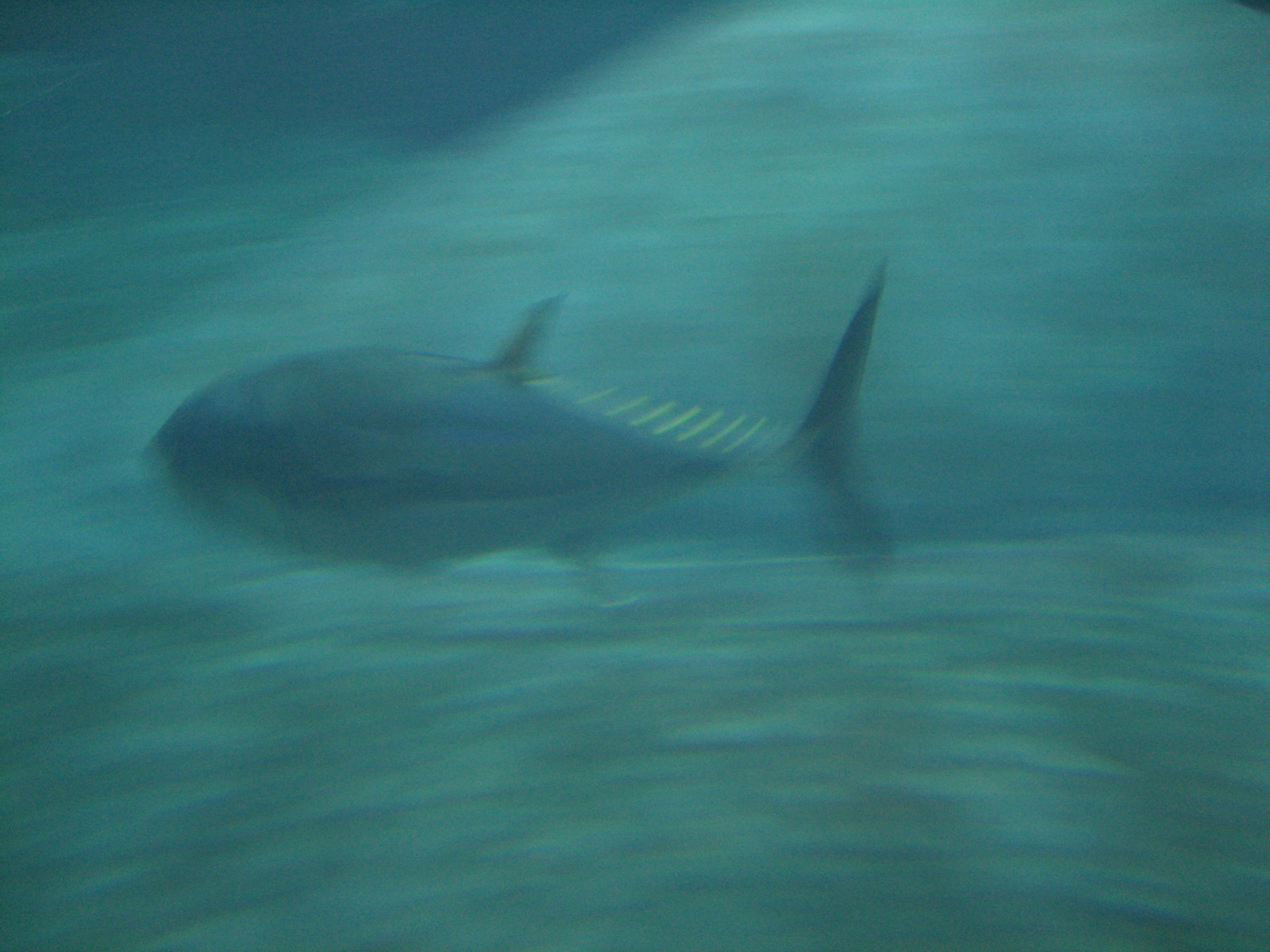This image is a very blurry underwater scene showcasing a large fish, possibly a yellowfin tuna, swimming away quickly. The photograph is taken from the left side of the fish, toward its back, so its head, eyes, and mouth are not visible. Instead, we can see its torso, dorsal fins, and tail with spiky barbs along the edges of the fins. The fish appears darker on the top, with a lighter underbelly. The water surrounding it is mainly turquoise, with a deeper turquoise shade near the surface in the top left corner of the image. The background is indistinct, with a potential sighting of a rocky area at the bottom, but no other fish, coral, or plants are visible due to the overall blurriness of the photograph. Despite the lack of clarity, the main takeaway is the fast-swimming fish, prominently identified by its serrated fin area.